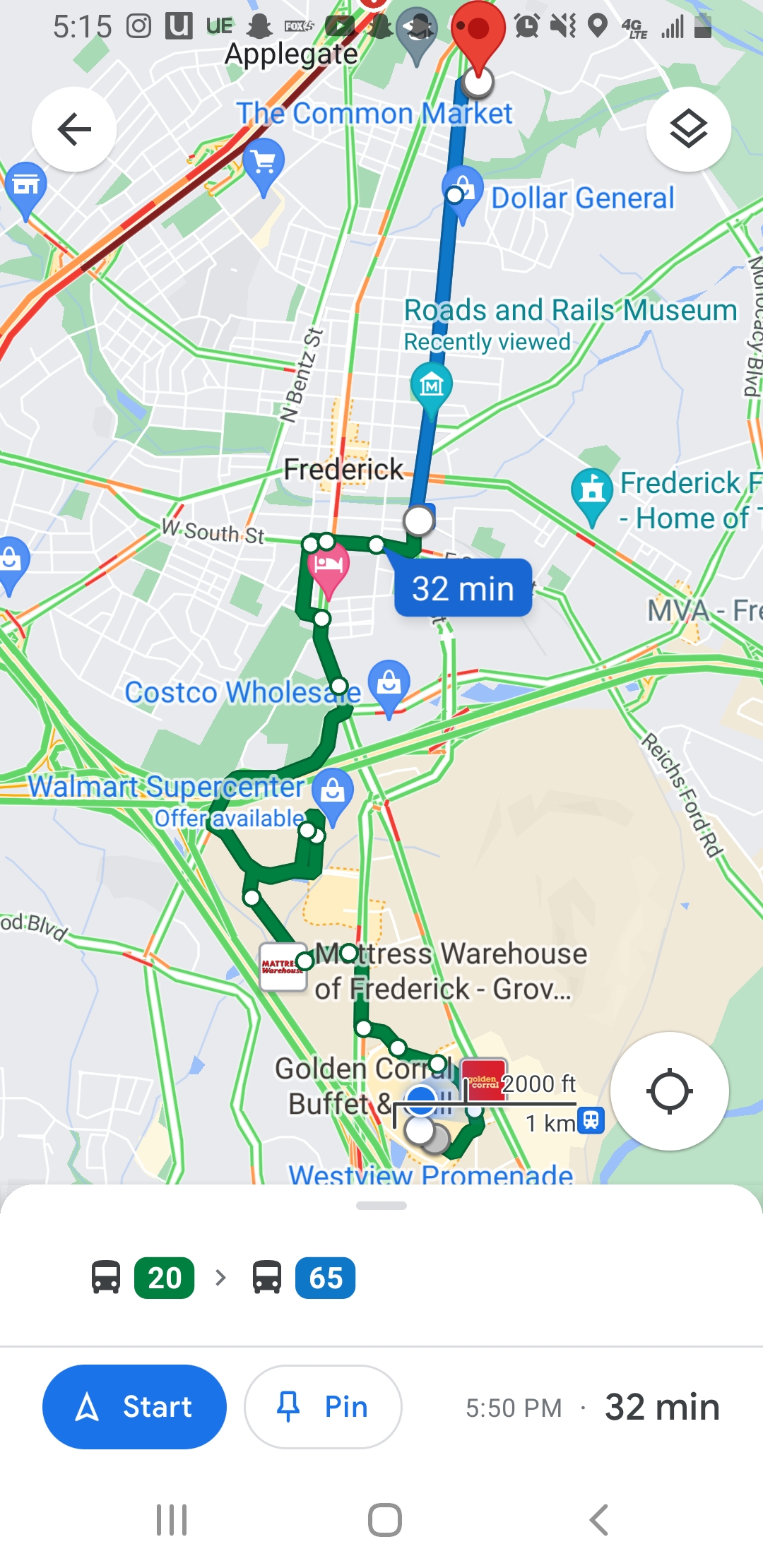This is a detailed screenshot of a Google Maps navigation on an Android phone, showcasing a route in Frederick, Maryland. The map highlights a journey starting at the Common Market, marked by a red pin, and ending at Westview Promenade. The path is visually represented with a blue line transitioning to green as it progresses. Key landmarks like Dollar General, Costco, Walmart, Golden Corral, Mattress Warehouse of Frederick, and Roads and Rails Museum are visible on the map. Notably, it indicates the travel time as 32 minutes and displays a time of 5:15 PM, with options like a "Start" button, a "Pin" button, and '2065' noted under Westview Promenade. The phone screen is at 50% battery with 4G connection, several app notifications including Snapchat, YouTube, Fox, Uber Eats, and Instagram, and a muted status with an unsnoozed alarm. The map's detailed elements, including road colors and clear markers, provide thorough navigation information.